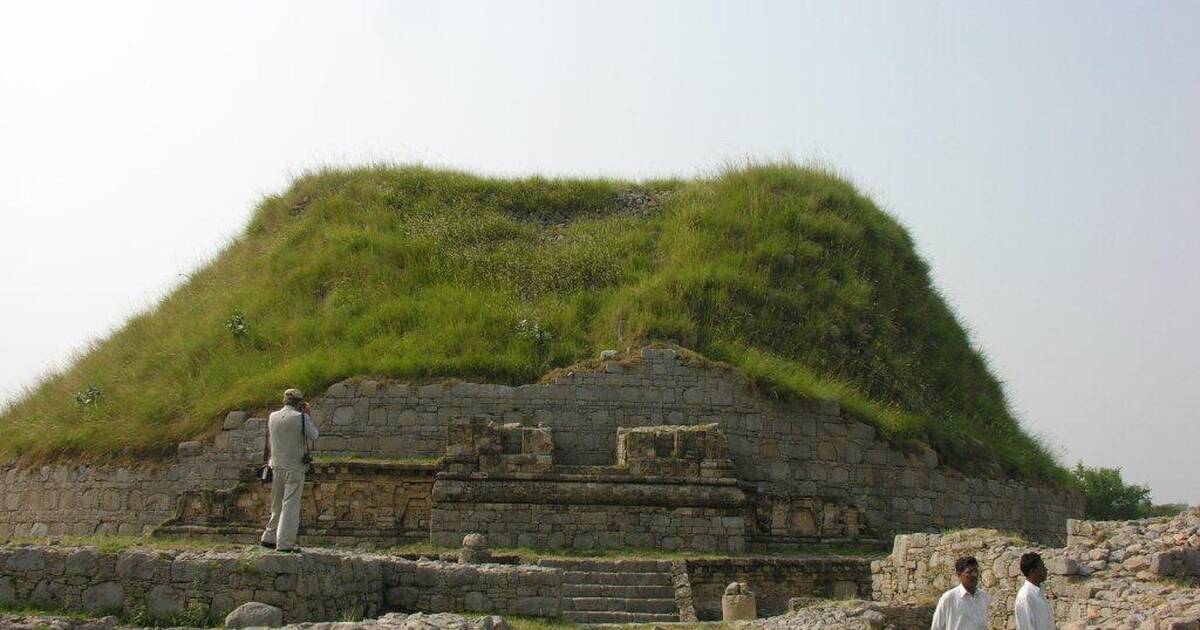This color photograph captures a historic tourist site featuring ancient ruins, likely a stupa and monastery, set in a foreign country. Central to the image is a sizable grassy mound or hill, indicative of a burial mound or a structure's remains. The mound is surrounded by a series of crumbled stone walls, which could be the foundation of a larger, bygone structure. Adjacent to these walls, there's a grassy platform reached by a short stone staircase of approximately six steps. 

The scene is animated by visitors: one man, slightly left of center, is engrossed in photographing the stone wall, while two other men dressed in white long sleeves are seen strolling towards the right, likely having just explored the site. The serene ambiance is complemented by a light blue sky, underscoring the area's historical gravity and tranquil beauty.